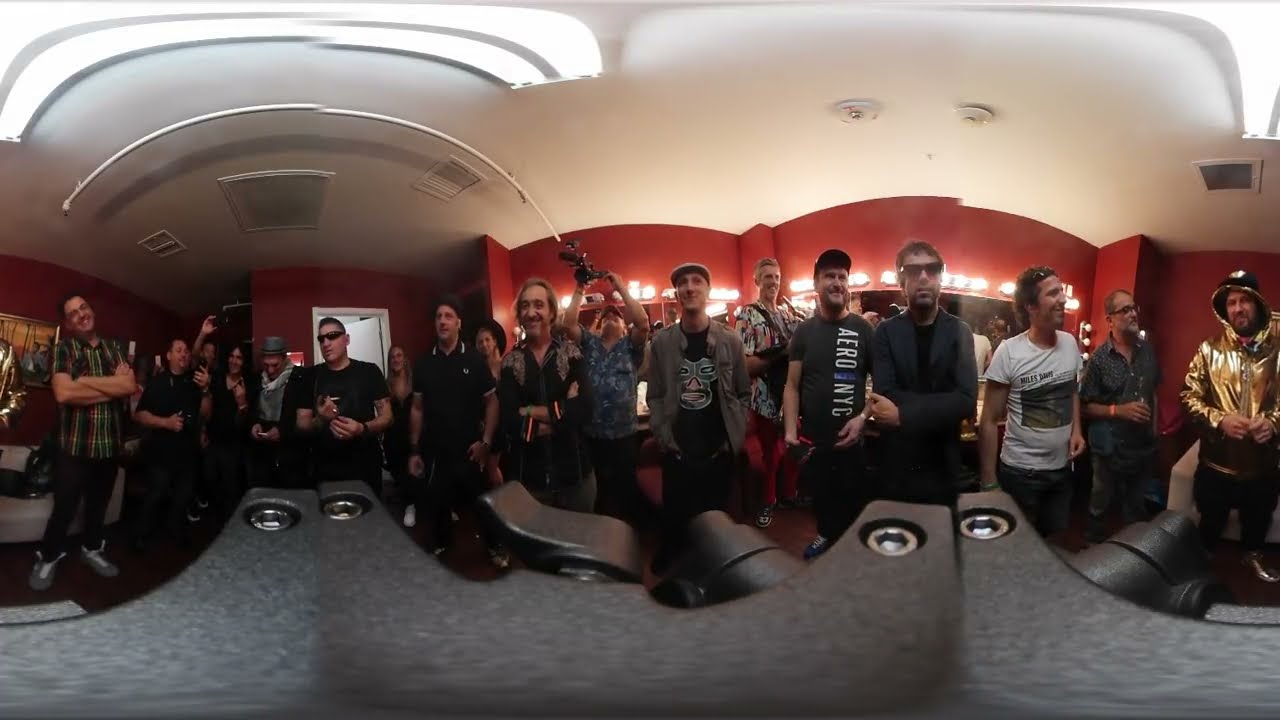The image depicts a lively, large room filled with approximately 40 to 50 people, predominantly men, gathered together, possibly for a social event or a casual party. Everyone is facing forward, with many smiling and interacting, creating an impression of a cheerful atmosphere. At the center of the group, a person is holding a camera, possibly capturing the moment. A variety of shirt colors are visible, including white, blue, black, gray, and some green. One person stands out in the crowd, partially cut off on the right side, wearing a glossy gold jacket and a helmet or hood, seen again in the left side creating a 360-degree effect.

The backdrop features a vibrant red wall adorned with shelves and white lights, reminiscent of a bar or a backstage area at a concert. Above, the ceiling is painted white. At the foreground’s bottom, there's a black object, likely a piece of plastic or a camera accessory, slightly blurring the lower edge of the image. The collective details, from the colorful attire to the red wall and white ceiling, contribute to a dynamic and engaging scene.